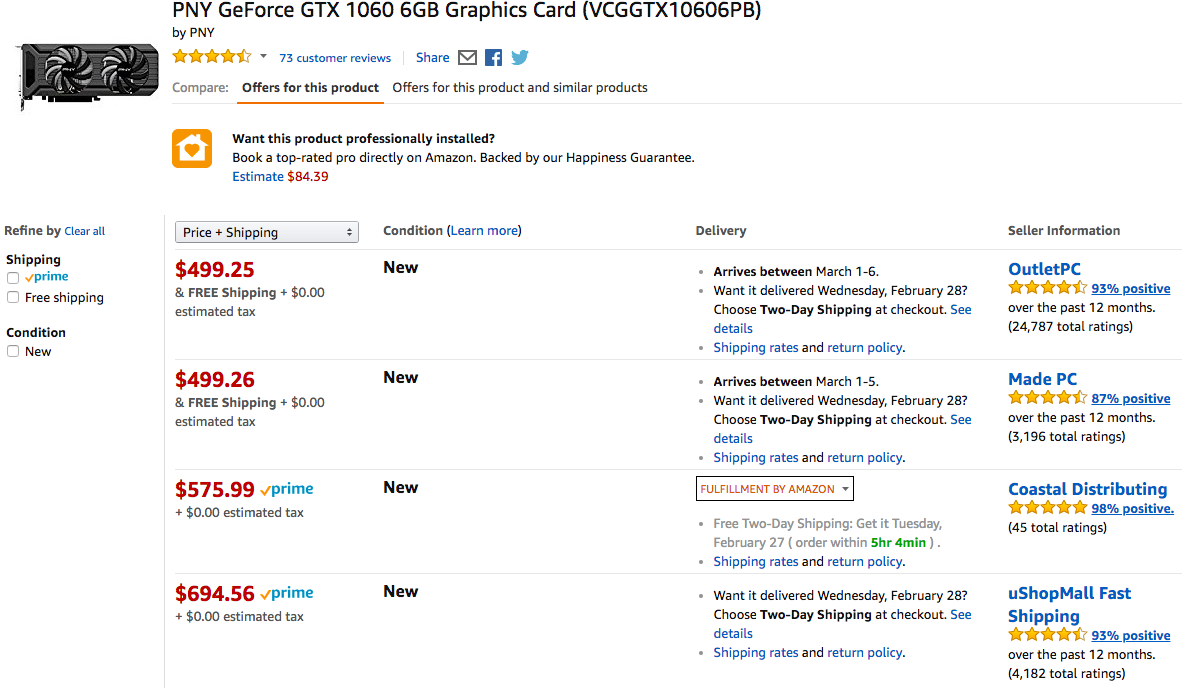This screenshot, taken from the Amazon website, showcases a computer product page focused on graphics cards. In the top left corner, it is evident that the user is viewing a specific product - the PNY GeForce XTX 1060 6GB Graphics Card. The main image of the graphics card reveals a black design with two visible cooling fans. Adjacent to the image, the product boasts a 4.5-star rating based on 73 customer reviews. Below the product details, several listings for the same model are displayed, each differing in price: $499.29, $499.26, $575.99, and $694.56. All listed items are in new condition. On the right side of the screen, additional information regarding delivery options and seller details can be seen, providing a comprehensive overview for potential buyers.